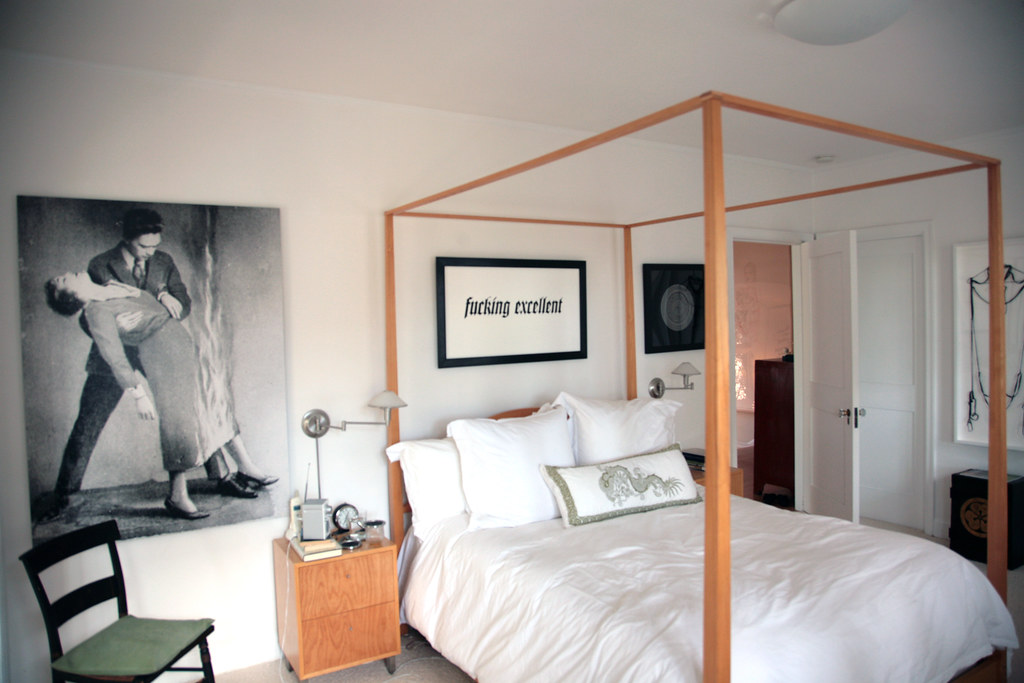This photograph captures a neatly arranged bedroom featuring a canopy-style bed frame made of tan-colored wood at each corner, extending up and across to form a simple overhead frame with no curtains. The bed is dressed in a pristine white comforter accompanied by four white pillows, with an additional white pillow featuring a green border and decorative design providing a touch of contrast. The room exudes a minimalist charm with its white walls, ceiling, and adjoining doors to the right.

The flooring is a warm tan-colored carpet. To the left of the bed, an oak or pine nightstand holds a sleek, silver swing-arm lamp. Adjacent to the nightstand, a dark brown chair with a green cushion adds a pop of color to the space. A black and white artwork adorns the wall, depicting a man in a suit holding a fainting woman, lending a classic vibe to the room. Above the bed, a black-framed picture boldly declares, "fucking excellent" in italicized black font, making a modern and striking statement.